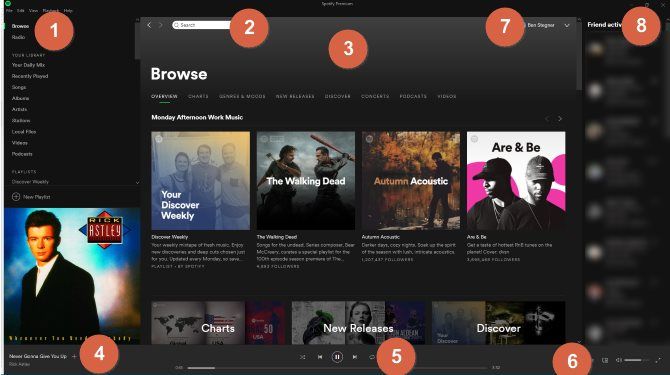The image appears to depict a music streaming or browsing website interface during a Monday afternoon session. The overall design features numerous small fonts that are challenging to read. The background of the site is black, with white text providing various labels and titles.

Prominently displayed on the screen are several red circles containing white numbers. These circles likely serve as navigation or selection markers and are arranged strategically across the interface. Starting from the top left, the circles are numbered and positioned as follows:
- No. 1: Top left corner
- No. 2: Towards the top right, adjacent to the first circle
- No. 3: Slightly lower than the second circle
- No. 4: Bottom left corner
- No. 5: Middle of the bottom edge
- No. 6: Near the right side, along the bottom edge
- No. 7: Above the sixth circle, closer to the right edge
- No. 8: Bottom right corner

The main sections of the website include options or playlist titles such as "Your Discovery Week," "The Walking Dead," "Autumn Acoustic," "R&B," "Charts," "New Releases," and "Discover." An album by an artist named "Astley" (spelled out as A-S-T-L-E-Y) is visible, although much of the surrounding text is blurred and difficult to read.

Overall, the visual cues and text suggest that the interface is dedicated to exploring and discovering new music, possibly guiding users through different playlists and new releases.